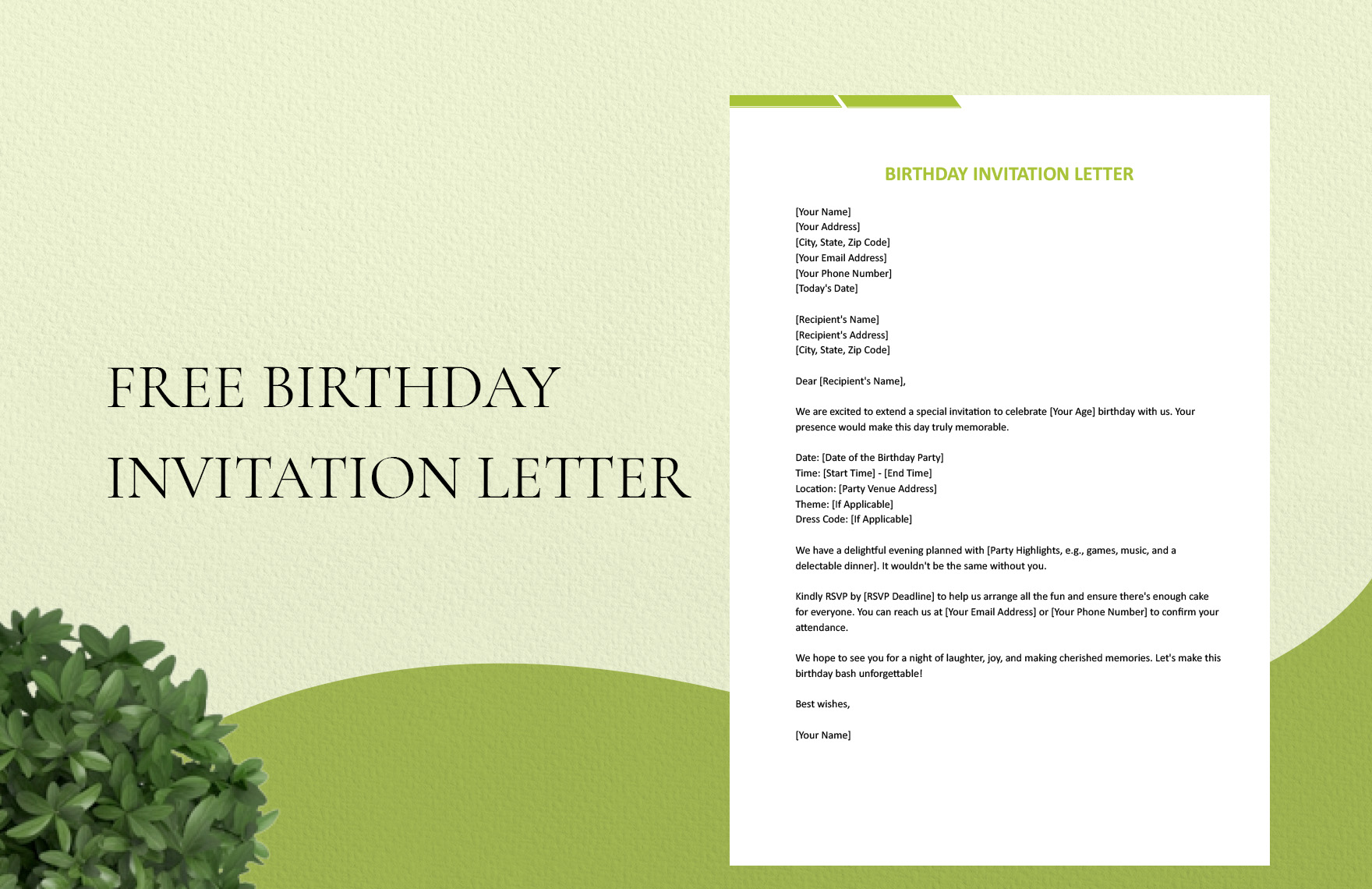The image depicts a free, printable birthday invitation letter template in a landscape layout. The design features a cream-colored background at the top, transitioning to a lime green section at the bottom. In the lower left-hand corner, leaves from a bush are visible, adding a touch of natural decor. On the left side of the template, bold black capitalized letters spell out "FREE BIRTHDAY INVITATION LETTER" across two lines. 

To the right, a sample invitation letter is displayed on a white backdrop with green headings. This template provides fields for the sender to enter various details: their name, address, email, phone number, the date, and the recipient's name and information. The sample text includes sections labeled for the occasion's specific details such as date, time, location, theme, and dress code, along with a prompt for the RSVP information. The letter concludes with a "Best wishes" message followed by a space for the sender to sign their name. This template serves as an easy and customizable solution for creating a personalized birthday invitation.